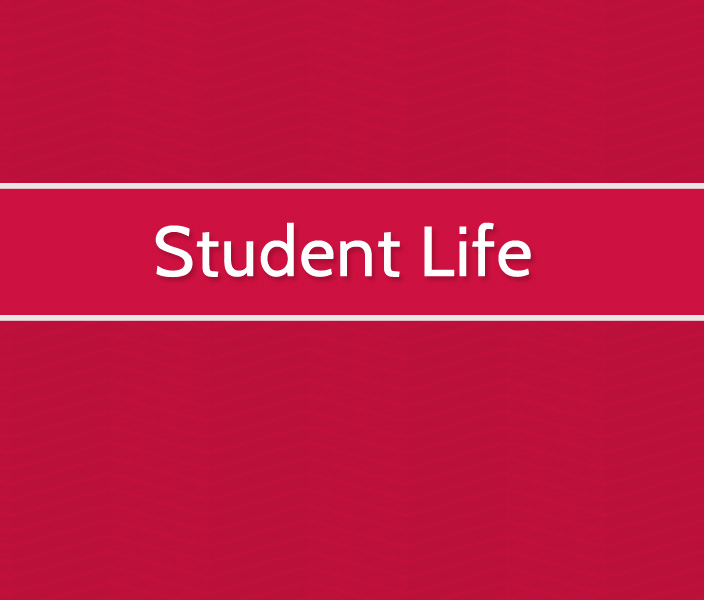The image features a slightly dark reddish background adorned with an inverted V-shaped white line pattern running horizontally across it. Near the upper middle section of the image, approximately six-tenths of the way up from the bottom, there is a prominent red banner bordered by thin white lines on the top and bottom. Inside this banner, centered in white text, are the words "Student Life," with the letters "S" and "L" capitalized and the rest in lowercase. The typeface is simple and unembellished, resembling Arial, with a font size estimated around 45 to 50 points. The white lines framing the text are thinner than the font size of the words. The overall presentation is minimalistic, evoking the look of an introductory slide in a presentation.